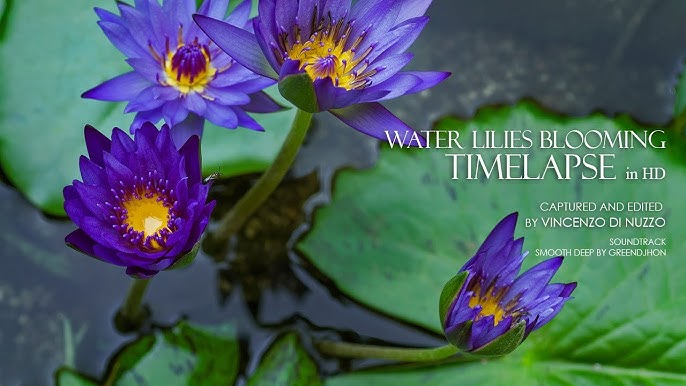The image showcases a captivating scene of purple water lilies in full bloom, accompanied by white, all-capital text that reads "WATER LILIES BLOOMING TIME-LAPSE IN HD." Below this, in smaller text, it mentions "captured and edited by Vincenzo Di Nuzzo" and "soundtrack Smooth Deep by Green Winner John." The scene features four prominent water lilies, each displaying vibrant purple petals with yellow inner leaves. The leftmost lily has a whitish-yellow center, while the two lilies in the middle have distinct purple centers. The lily on the far right is turned slightly, obscuring its center from view. Beneath these striking flowers, lush green lily pads float serenely on the water, adding to the image's natural beauty.